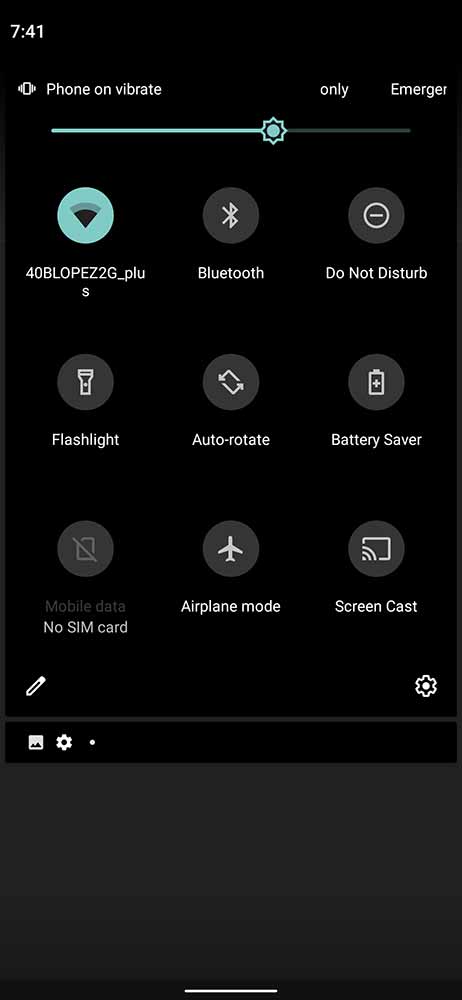This image, captured as a screenshot from an Android cellphone, displays the quick settings panel opened by swiping down from the top of the screen. The panel reveals nine different icons arranged in a 3x3 grid, offering various settings and features for the user to quickly access.

From left to right, the top row includes the Wi-Fi option, the Bluetooth option, and the Do Not Disturb button. The second row, also left to right, features the Flashlight option, the Auto-Rotate feature, and the Battery Saver button. The final row contains the Mobile Data button, the Airplane Mode option, and the Screencast button.

In the upper left-hand corner of the screen, the time is displayed as 7:41 AM/PM, accompanied by a vibrate icon indicating that the phone is set to vibration mode. Below the time and vibrate icon, a brightness slider allows the user to adjust the screen brightness. The interface design is functional and user-friendly, enabling efficient access to commonly-used settings and features.